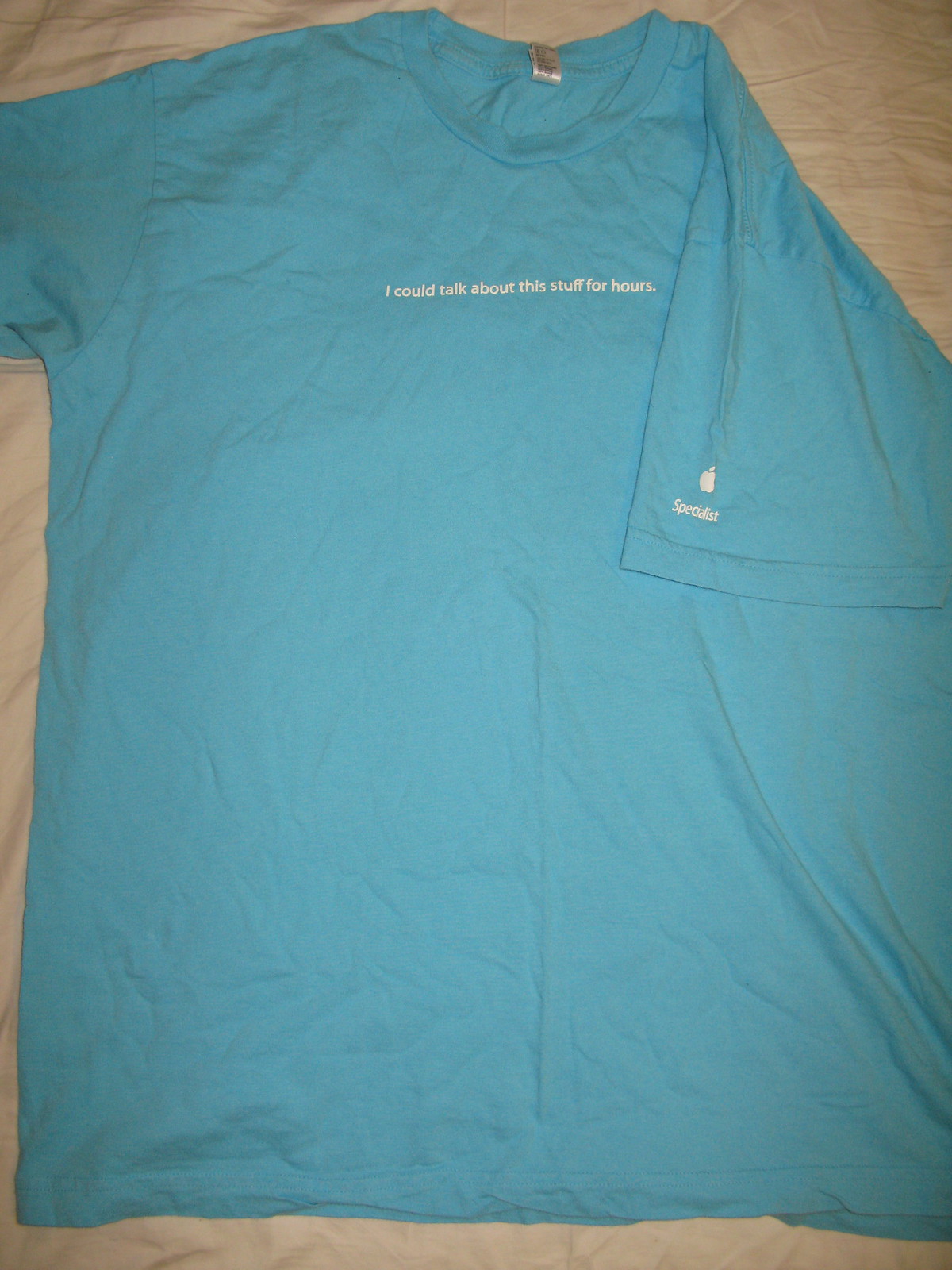A light blue short-sleeve t-shirt is laid out on an off-white fabric surface. The shirt features tiny white text positioned on the upper chest area. The left sleeve is folded over from the shoulder down to the chest, displaying a small white emblem with matching white text on the back side of the folded sleeve. The round collar of the shirt includes a white rectangular care tag at the center of the back. Noticeable wrinkling is present on the shirt, especially on the right side, indicating it was not laid out smoothly.